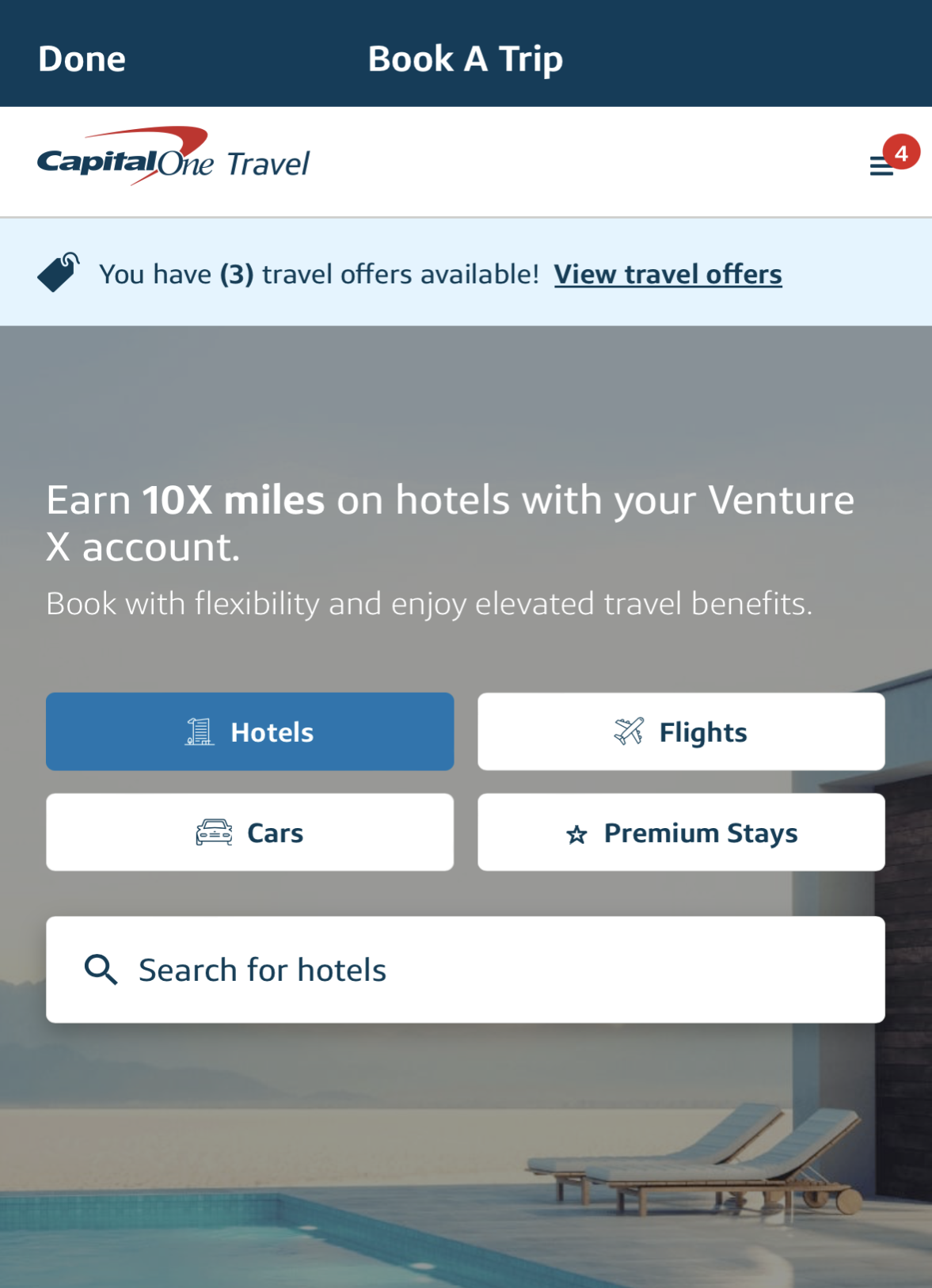**Caption:**

The image is a screenshot of the Capital One Travel website's "Book a Trip" page in portrait mode. At the top, there is a dark blue bar with centered white text reading "Book a Trip," and to the left, it says "Done." Below, a white bar displays the Capital One logo with the red swoosh and the text "Capital One Travel." To the right of this bar, there is a menu icon (three stacked lines) with a red circle overlay containing a white number "4."

Following this, a light blue bar with dark blue text and a luggage tag icon indicates, "You have (3) travel offers available! View travel offers," with "View travel offers" underlined as a hyperlink.

The remainder of the screen features a photographic background of empty chaise lounges arranged by what appears to be a luxury pool, possibly indoors. The setting looks high-end with a blue-gray wall behind the pool.

Overlaying the photo, large bold text states, "Earn 10x miles on hotels with your Venture X account," and in smaller text, "Book with flexibility and enjoy elevated travel benefits." Underneath this text, there are three rows of options and search functionalities:

1. The first row includes two buttons labeled "Hotels" (highlighted in blue with a building icon) and "Flights" (white with an airplane icon).
2. The second row consists of "Cars" (white with a car icon) and "Premium Stays" (white with a star icon).
3. The third row features a search bar with a magnifying glass icon, labeled "Search for hotels."

The overall design is visually appealing and user-friendly, aiming to facilitate booking travel with added benefits for Capital One Venture X account holders.